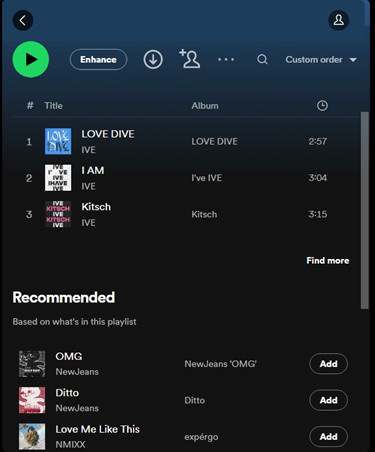The image depicts a partial screenshot of a mobile phone interface showcasing a music player application. At the top left, there is a prominent green play button, followed by a button labeled "Enhance" to its right. Below these, there is a downward arrow icon, indicating a dropdown menu. Further to the right is an icon representing a user with a plus sign, leading into a search bar. Adjacent to the search bar, the words "Custom Order" are visible, suggesting a dropdown menu for sorting options.

The interface is split into three main columns labeled "Title," "Album," and "Time," with a clock symbol next to the "Time" column. The first song listed is "Love Dive" by IVE with a duration of 2 minutes and 57 seconds. The second song is "I AM" by IVE, lasting 3 minutes. The third listed track is "Kitch" by IVE, with a runtime of 3 minutes and 15 seconds.

Beneath the listed songs, the application recommends additional tracks: "OMG" by New Jeans, "Ditto" by New Jeans, and "Love Me Like This" by NMIXX, suggesting these songs can be added to the playlist.